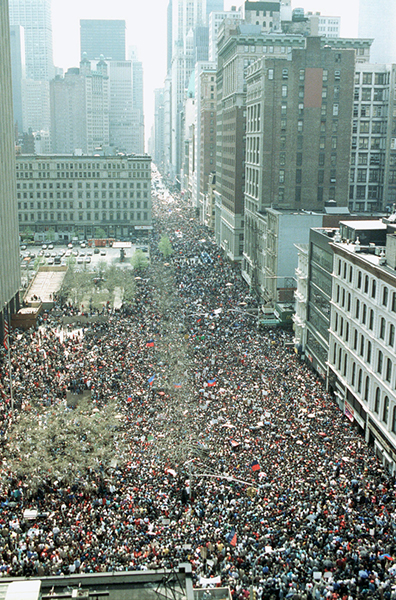This color photograph captures an incredibly dense street scene in a large city, possibly New York. Taken from several stories up, the aerial view provides an expansive look across an avenue teeming with people—hundreds of them filling both the street and the sidewalks. Even the rooftops are populated, highlighting the overwhelming turnout for what appears to be a major event, possibly an outdoor concert, demonstration, or holiday celebration. The cityscape includes tall buildings whose rooftops have visible generators, and some are so tall that their tops aren't even in the frame. Notably, there’s an individual in a red jacket or shirt perched atop a street light. Off to the left-hand side, an American flag waves, adding a patriotic touch to the bustling urban tableau. The overall scene is chaotic yet vibrant, capturing the essence of a city throbbing with human activity and leaving no space for cars in what is usually a busy thoroughfare.